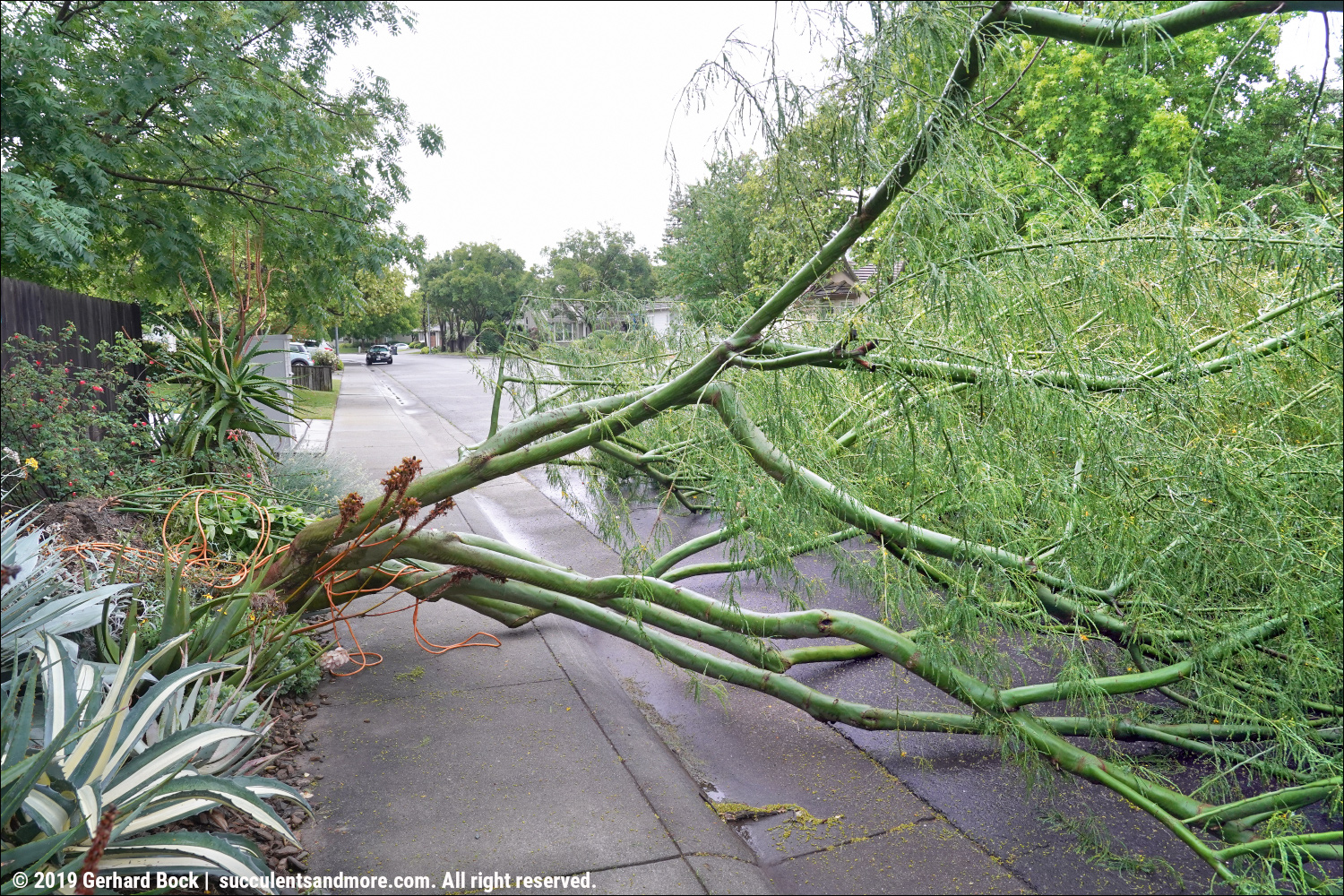This landscape photo captures a fallen tree sprawled across a suburban street amidst a lush, green neighborhood. The tree, with its green leaves and branches, appears to have toppled from a garden bed on the left side of the road, possibly due to a recent storm as the ground is wet. The street, lined with greenery and some small plants, features a dark gray asphalt surface with a residential sidewalk running beside it. A wooden fence and an electricity box are partially visible behind the garden bed. In the background, a dark car and another vehicle are parked along the street. There are also orange cords wrapped around the base of the tree, the purpose of which is unclear. The image is copyrighted, bearing the mark "2019 Gerhard Bock, succulentsandmore.com, all rights reserved." The sky above is white, and there are no visible buildings or people, giving the scene a tranquil and somewhat isolated feel.